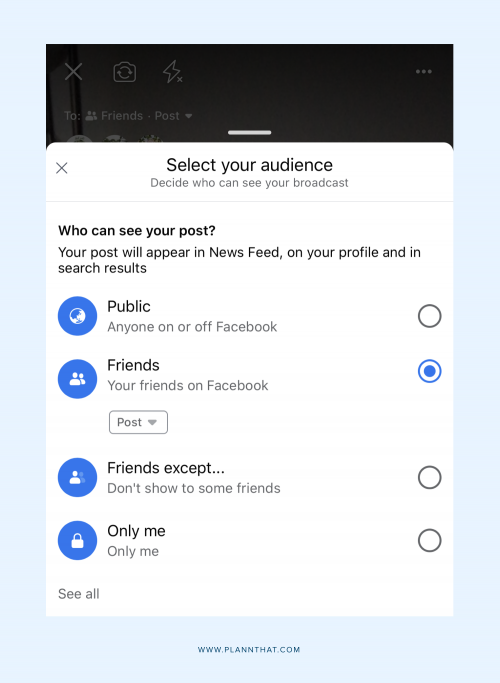This image depicts a screenshot from an unidentified social media platform. At the top of the screen, there is a black horizontal bar. Below this bar, a white pop-up window appears, occupying the central part of the screen. The pop-up window's title reads "Select Your Audience." Beneath the title, a prompt states: "Decide who can see your broadcast." Below the prompt, multiple audience selection options are listed, allowing users to choose between making their broadcast visible to "Public," "Friends Only," "Friends Except," or "Only Me." These settings enable users to control the visibility of their content on this platform.